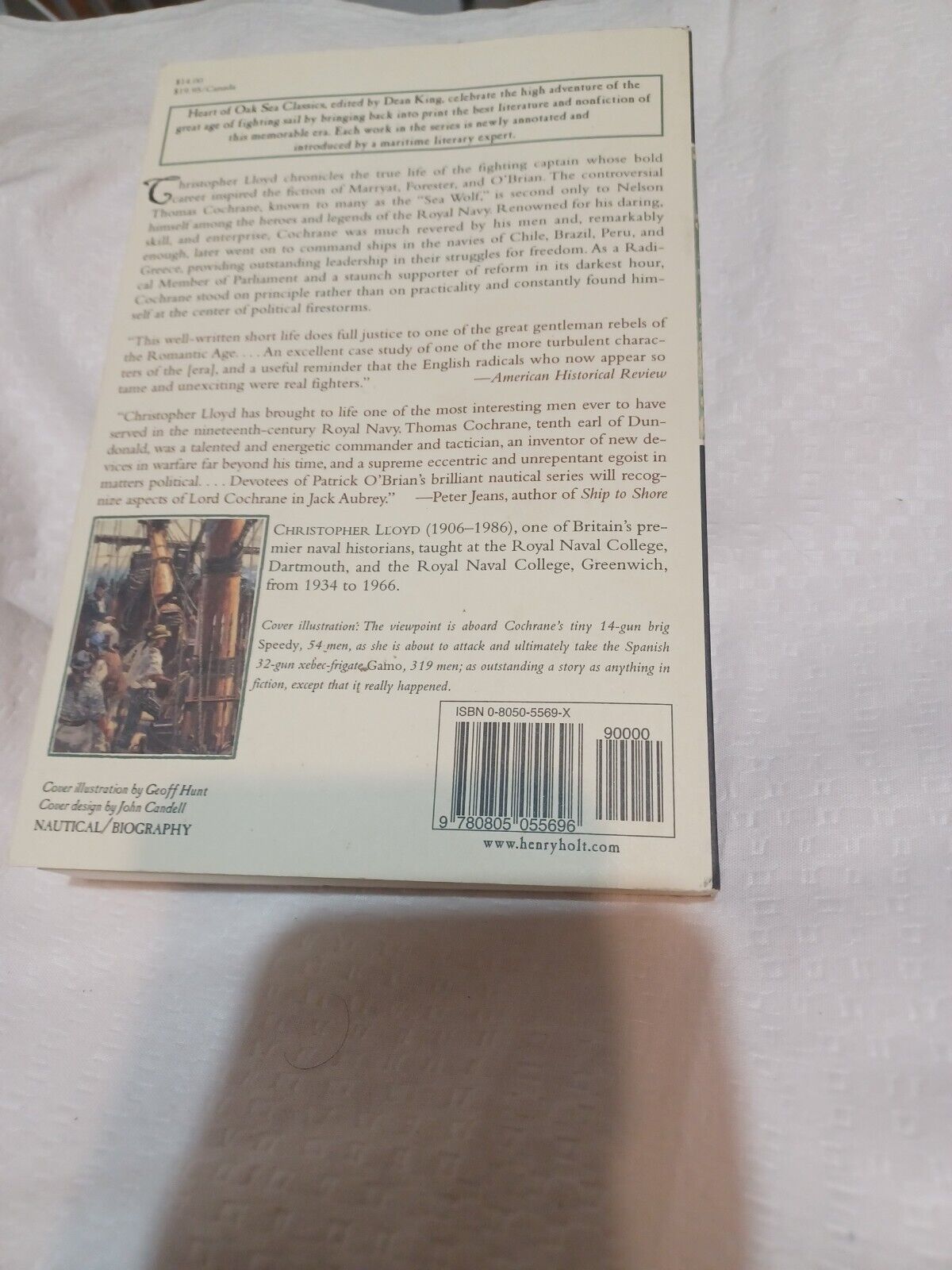The back cover of this book, which could be either a hardcover or paperback, is presented against a white sheet or similar material. The cover features a summary, though the tiny print makes it hard to read. The content appears to provide a detailed look into the life of Thomas Cochrane, the 10th Earl of Dundonald, renowned for his contributions to 19th-century Royal Navy tactics and inventions. Despite some blur, it mentions a review from the American Historical Review, praising the book for bringing to life this notable historical figure, authored by Christopher Lloyd. The cover includes a website (www.henryholt.com) and has text filling most of the space, accompanied by a small image in the lower left corner, partially obscured by a shadow likely cast during the image capture.